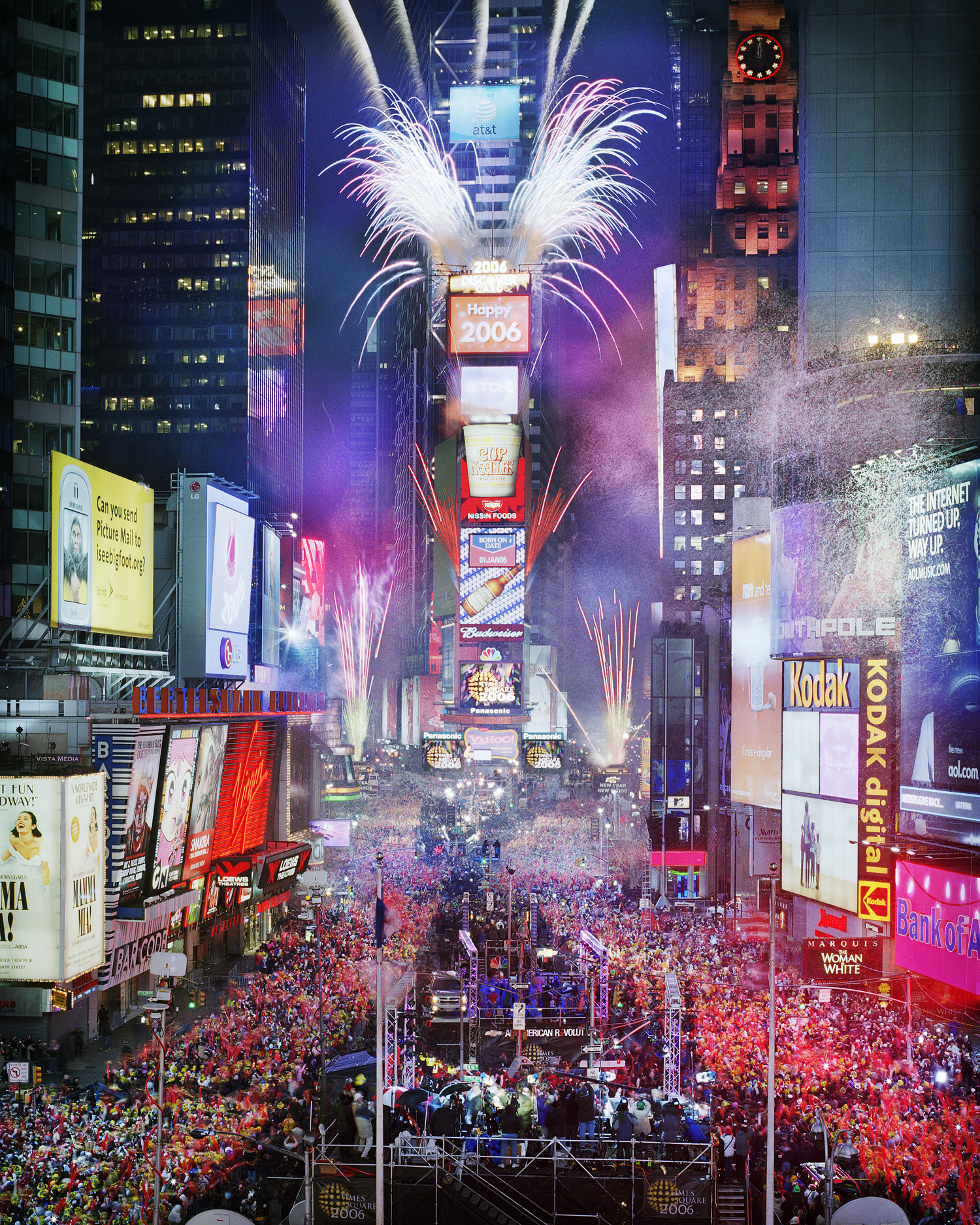This photograph captures the vibrant energy of Times Square in New York City during the New Year's Eve celebration in 2006. Taken from a high vantage point in portrait orientation, the image showcases the iconic skyline with towering skyscrapers lining both sides. In the center background, a prominent tower features a red marquee at its pinnacle displaying "Happy 2006," from which dazzling fireworks erupt against the night sky. The lower section of the frame is dominated by the luminous billboards of Broadway, illuminating the dense crowds below. Thousands of jubilant revelers are crammed together, surrounding an elevated metal frame stage situated prominently in the middle foreground, where live performances are taking place. The air is thick with celebratory smoke, particularly noticeable to the right, dispersing amidst the spectacular fireworks and confetti showering down over the jubilant mass.